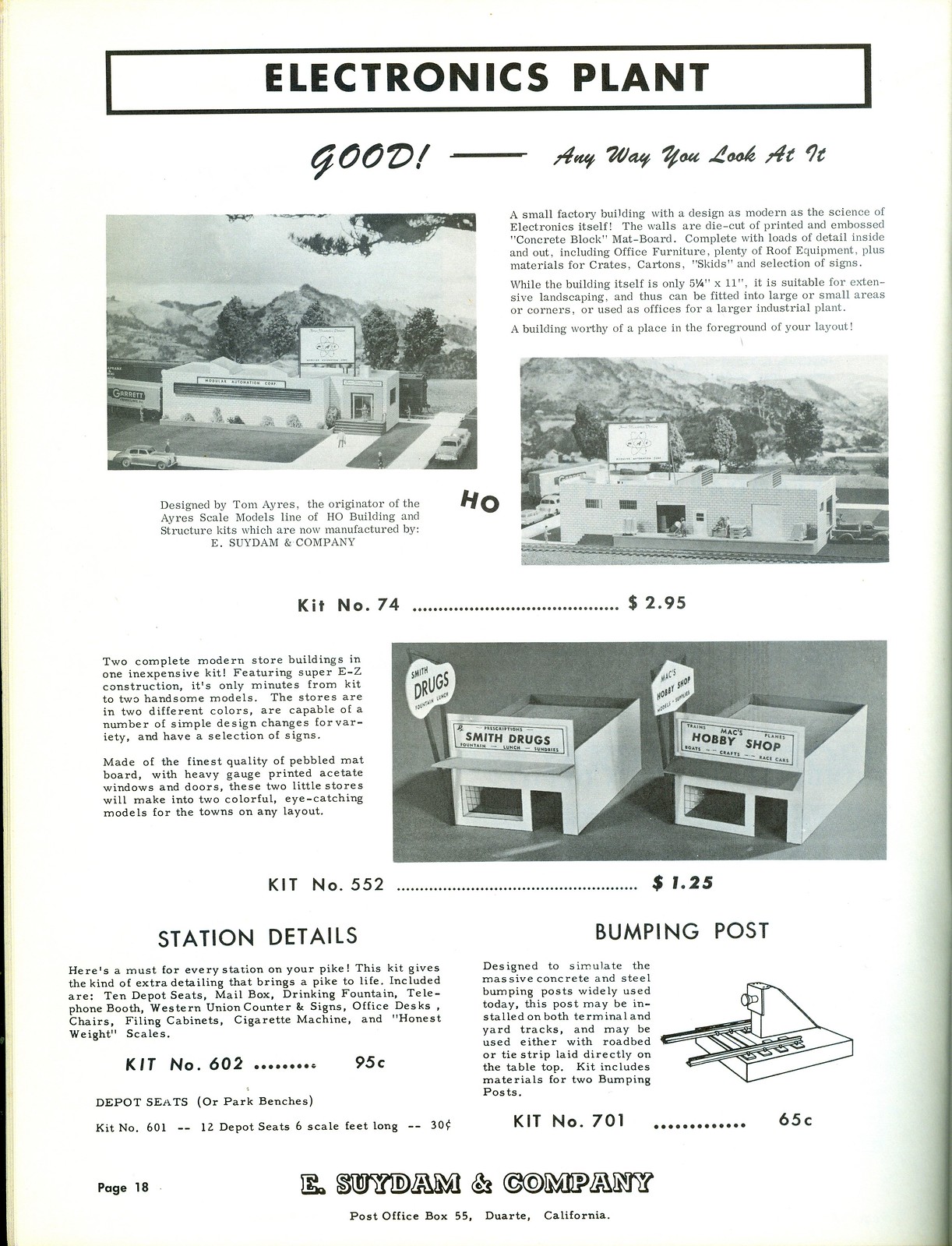The rectangular image is an aged, yellowed magazine advertisement, possibly from a brochure or ordering catalog, featuring black-and-white photographs of small-scale model buildings designed for architectural purposes. The bold, black title at the top reads "Electronics Plant" with the tagline "Good, any way you look at it" beneath it. Scattered across the page are several photographs displaying different model kits available for purchase. The first kit, shown in two images depicting various angles, is listed as Kit Number 74 for $2.95. Following this, two smaller identical models are labeled as Kit Number 552, priced at $1.25 each, with signs identifying them as a Hobby Shop and Smith Drugs, respectively. Below these, additional details about "Station Details" and "Bumping Post" kits are provided, with Kit Number 602 available for $0.95 and Kit Number 701 for $0.65. The bottom of the page features the company's name, E. Suydam and Company, along with their contact address: Post Office Box 55, Duarte, California.